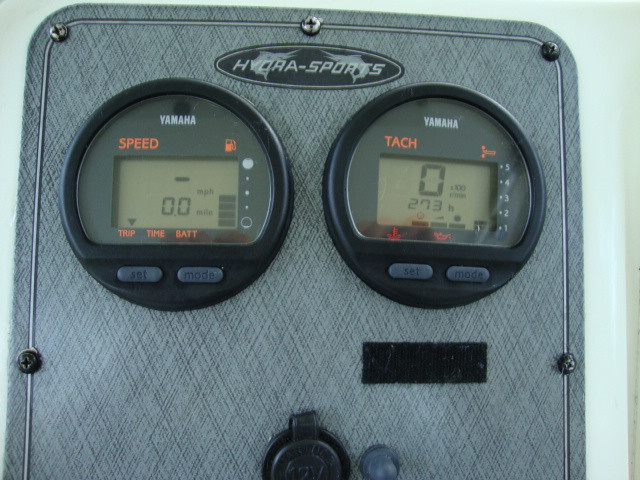This color photograph captures a detailed close-up of a jet ski's control panel, predominantly featuring a gray-white, crisscross-patterned, rectangular trim plate. The image is square in shape. Prominently displayed on the upper half of the trim plate are two main dials, both round and primarily black, with sunken glass bezels.

At the top of the trim plate, an elliptical emblem with a black background is adorned with two bluefin fish facing each other and the word "HYDROSPORTS" in bold, white, uppercase letters. 

Both dials feature the brand "YAMAHA" in bright orange at the top. The left dial, labeled "SPEED," includes a gas pump icon, indicating its function as a speedometer with a fuel gauge. The right dial, labeled "TACH" in uppercase letters, likely serves as the tachometer. Below these labels, each dial has two small, elliptical buttons marked "SET" and "MODE."

Additionally, below the right dial, there is a small rectangular display, possibly used for additional readouts or settings. The meticulous design of this control panel highlights the advanced functionality and attention to detail typical of a high-performance jet ski.